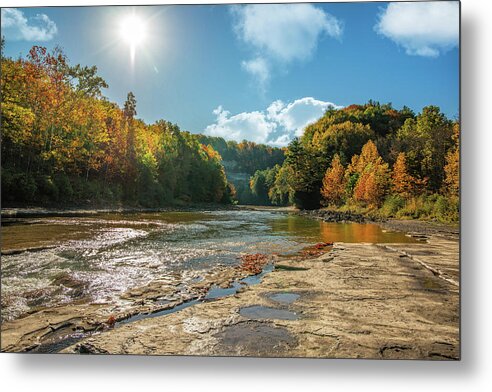This photograph captures a serene wilderness scene, likely located in a national park or the backcountry of the Pacific Northwest or Canada. The foreground features saturated mudflats, colored in shades of brown and red, interspersed with small streams of water and occasional footprints. These mudflats lead into a shallow, green-hued river, its banks flanked by rocky shores and accented by low flat rocks, some of which are exposed due to the low water level. Tall, majestic evergreen trees, in an array of autumnal colors including greens, oranges, reds, and yellows, line either side of the river. The sky above is a bright blue, dotted with light, wispy cumulus clouds. The sun beams down brightly from just above the horizon, casting its rays on the landscape, its light reflected in the river and against the mudflats. In the distance, the valley becomes obscured by more towering trees, creating an enchanting backdrop. Overall, the sunlight is drying out parts of the ground, causing some areas to crack, yet it brings out the vivid colors of the autumn foliage and illuminates this picturesque natural scene.